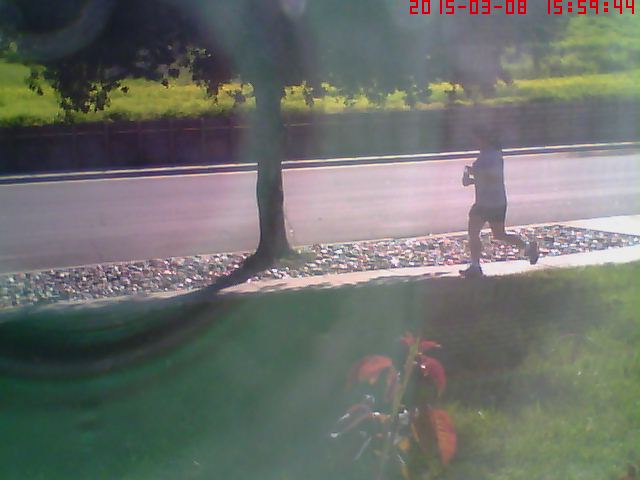In this vibrant image, captured on March 8, 2015, at 3:54 PM, a person is seen running on a sunlit sidewalk bordered by a lawn of lush green grass. The runner is framed by a path edged with decorative rocks that enhance the landscape design. A prominent tree stands by the sidewalk, casting a soothing shade over much of the verdant lawn. Beyond the tree, the scene extends to a road, across which stands a fence guarding either a hedge or a field abundant with grass or flowers. Adding to the scene's detailed beauty, a rose bush, with its delicate stem and branch, graces the foreground.